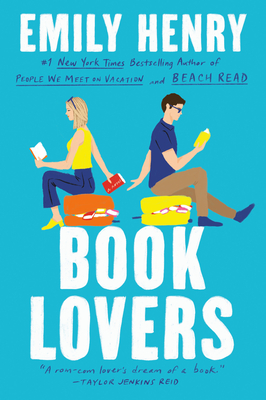The cover of the book features a solid medium-to-teal blue background. At the top, "Emily Henry" is prominently displayed in large white font. Below, in smaller dark blue font, it reads "Number one New York Times bestselling author of People We Meet on Vacation and Beach Read." Dominating the center of the cover, the title "Book Lovers" is written in giant white font. Underneath that, in dark blue font again, is a quote: "A Rom-Com Lover's Dream of a Book - Taylor Jenkins Reid." The illustrations show a white woman and a white man sitting back-to-back on cushions that look like sandwiches, each absorbed in a book. The woman, with blonde hair, is wearing a yellow shirt and blue pants, and she is seated on an orange cushion. The man, with brown hair, wears a blue shirt and khaki pants, sitting on a yellow cushion. The woman is reaching behind her to hand the man a red book, suggesting a connection despite their apparent focus on their own reading. The overall design contrasts the vibrant yellow and orange elements against the predominantly blue background.